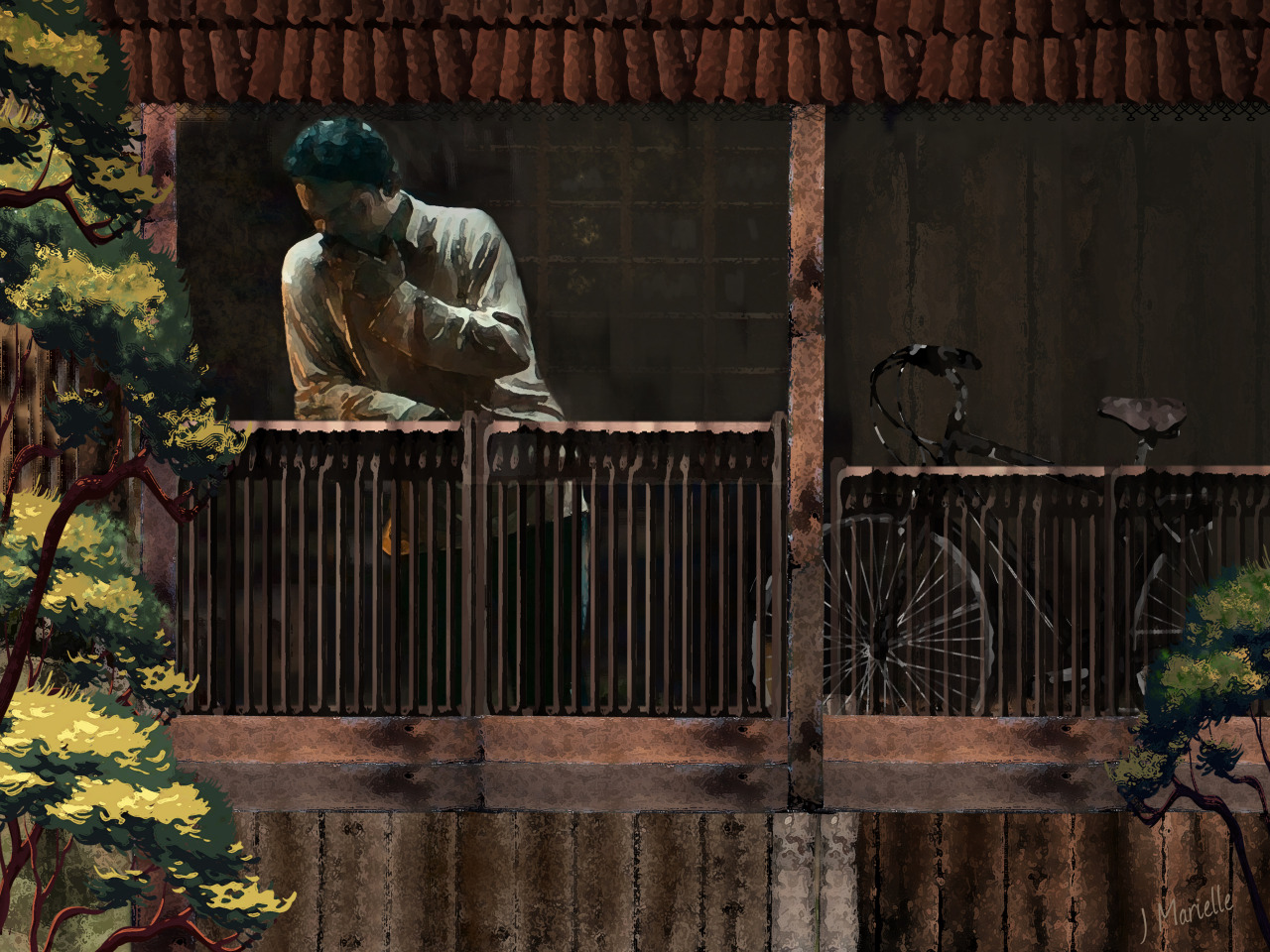This detailed painting, with an artist's signature "Che Marielle" in the lower right-hand corner, portrays a scene with rich elements. The focal point is a man of darker skin tone standing on a wooden balcony, partially covered by a roof. He has black, short hair and is dressed in a beige shirt or a white to gray long-sleeved, collared shirt, and dark pants. The man, who appears to be in deep contemplation, has his hand to his chin while leaning against the railing made of thin wooden slats. Adjacent to him, on the right side of the balcony, leans a black bicycle with a beige seat.

Below the balcony, the structure reveals vertically aligned wooden slats. The scene is further enhanced by natural elements, including a flowering tree on the left side and another smaller tree on the right. Bushes have grown up on the left side, adding greenery that reaches the height of the balcony. This mixed-media painting, with an impressionistic style on the man, captures a moment of reflective thought in a serene setting.